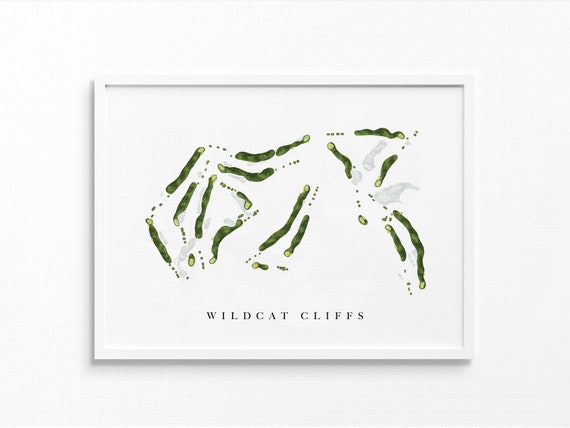The image is a highly minimalist photograph capturing a white framed poster against a stark white wall. The poster itself is predominantly white, embedding a faintly abstract, hand-painted or drawn image that appears to depict an aerial view of green, worm-like shapes arranged in various formations. These formations might represent cliff formations known as "Wildcat Cliffs," as indicated by the text centrally placed about two inches from the bottom of the poster in all capitalized, gray serif font. The green shapes are dispersed across the poster with a set of two in the middle, a triangular arrangement of three in the upper right, and multiple clustered on the left, suggesting an artistic interpretation of an aerial landscape. The entire composition exudes a clean, fresh, and intriguing aesthetic, blending elements of abstract art with hints of geographic or natural imagery, evoking both the impression of cliff formations and perhaps a semblance of islands floating in a sea.